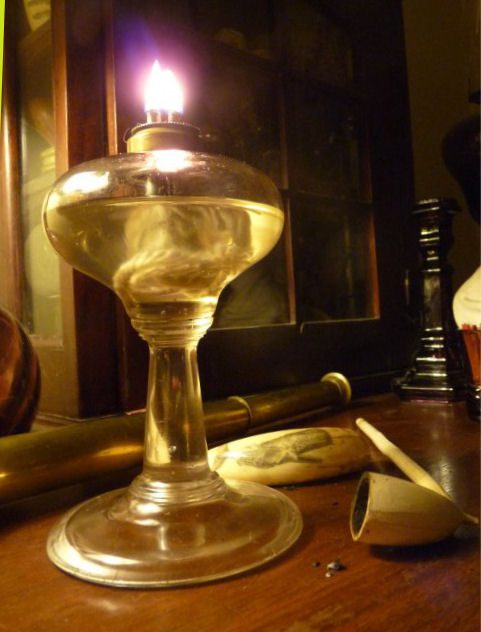The image depicts a vintage setting in a dimly lit room featuring an old-fashioned oil lamp prominently displayed on a redwood table. The oil lamp, an antique piece, has a round glass base filled with a flammable liquid and a thick cotton wick emerging from it, glowing with a steady flame. Next to the lamp lies an age-old tobacco pipe, a testament to the historical ambiance of the scene. Adding to the collection of antiquities, there's a candlestick and a golden spyglass-like cylinder, extending about halfway along the table. In the background, a large wooden hutch with glass-paneled doors stands majestically, housing more vintage treasures. This vignette is richly detailed, evoking a sense of nostalgia and timelessness.